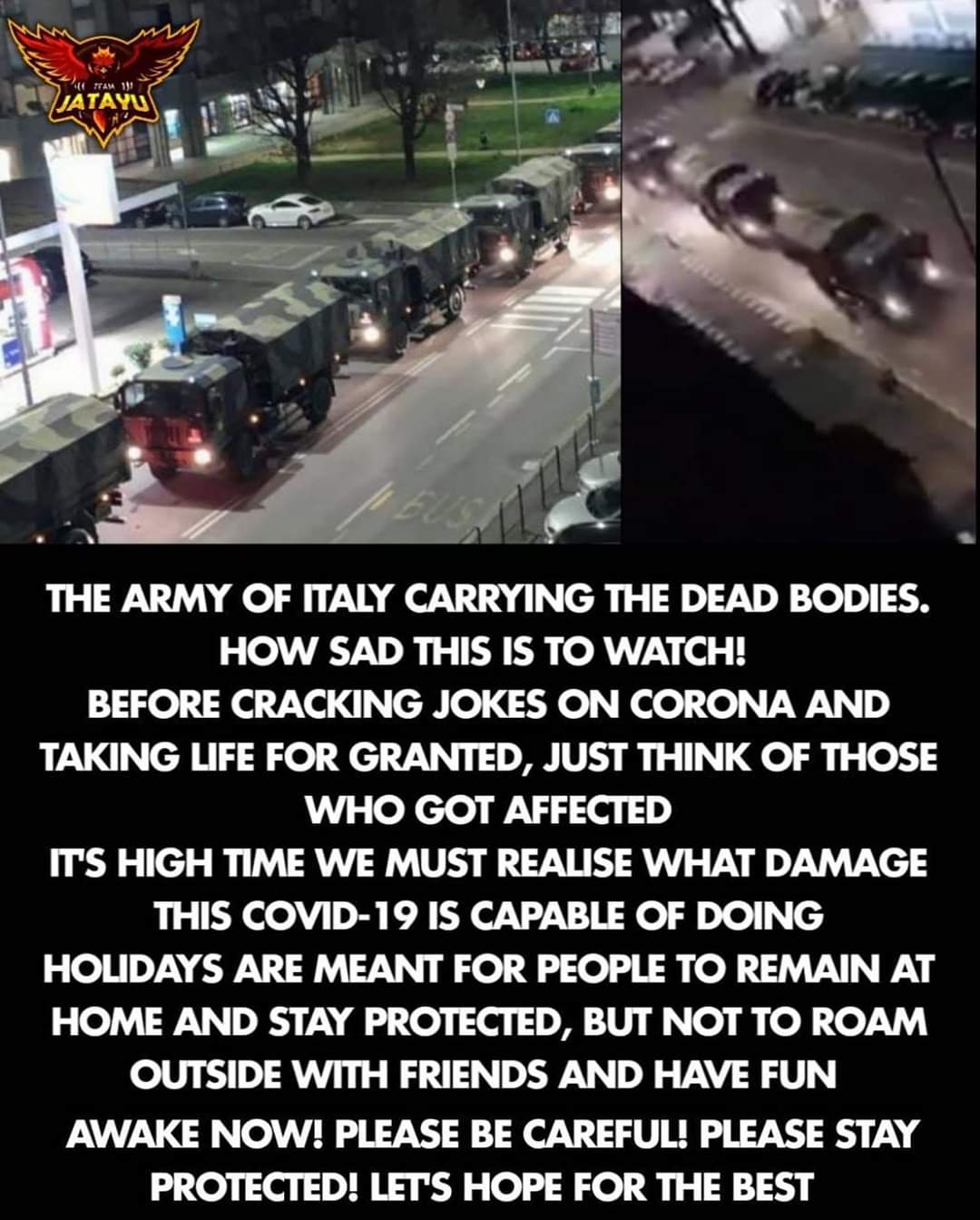This collage image is a vertically aligned rectangle featuring two photographs at the top and centered white text on a black background at the bottom. The text is in all caps and contains an important message about the impact of COVID-19. 

In the upper left corner, there's a small picture of several military trucks driving down a regular street at night, their headlights illuminating the scene. The surroundings feature grassy lawns, trees, and a few buildings. A logo labeled "J-A-T-A-Y-U," with red wings and gold letters, sits in the upper left of this image. To the right, a somewhat blurry photograph, possibly from a traffic camera, offers a top view of the same convoy of trucks on the same street.

The white text below reads: "The Army of Italy carrying the dead bodies. How sad this is to watch. Before cracking jokes on Corona and taking life for granted, just think of those who got affected. It's high time we must realize what damage this COVID-19 is capable of doing. Holidays are meant for people to remain at home and stay protected, but not to roam outside with friends and have fun. Awake now. Please be careful. Please stay protected. Let's hope for the best."